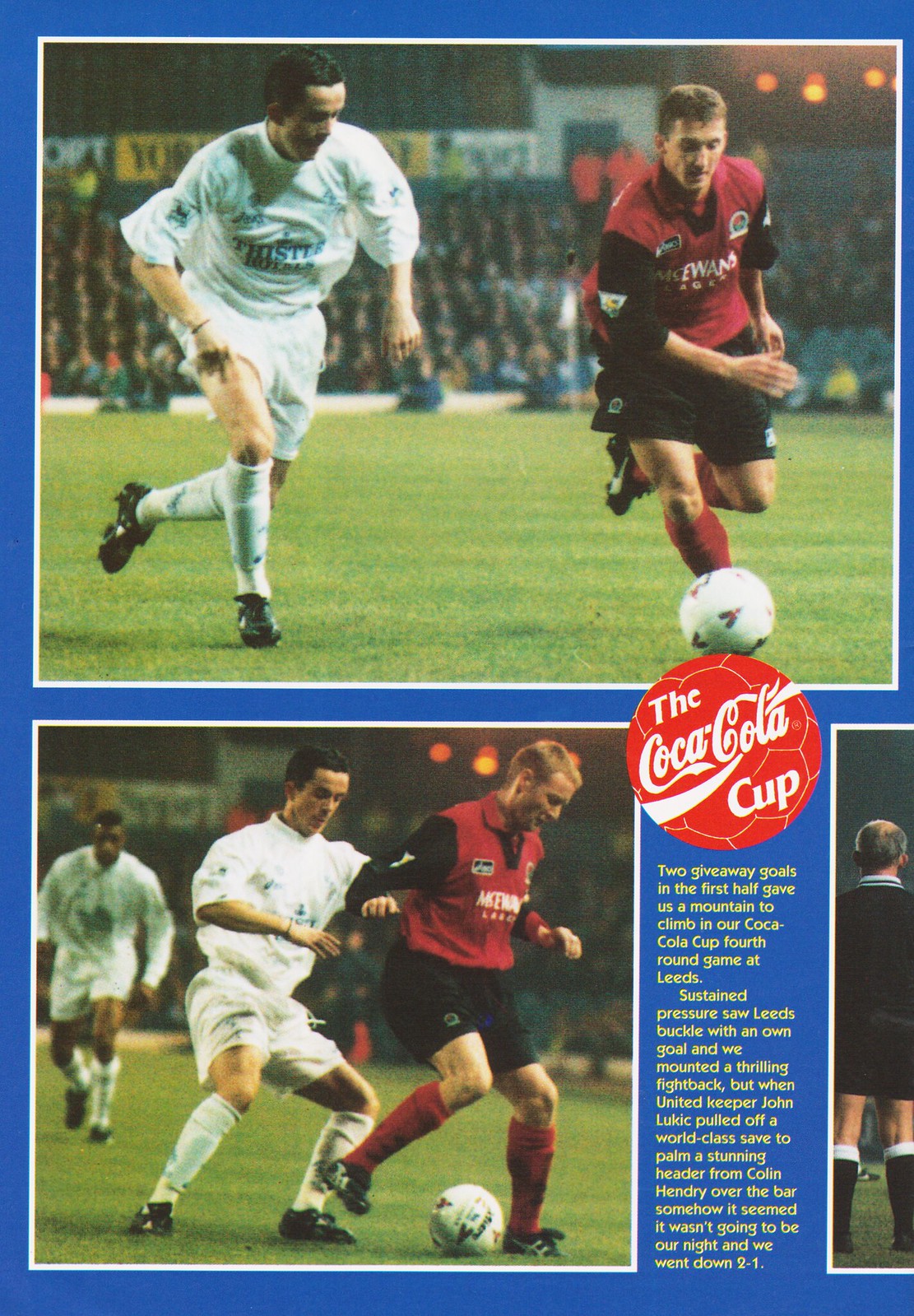The image appears to be a page from a sports magazine or program, framed in blue. It features a detailed depiction of a soccer match, with the majority of the page taken up by two large, vividly colored photographs. The top photo shows two soccer players on a field with green grass and packed stadium stands in the background. The player on the left, wearing a white jersey with black shoes, has dark hair. The player on the right, dressed in a red and black sports outfit, has lighter brown hair and is poised to kick a soccer ball on the ground. 

Below this image, on the left, a second photograph captures the same two players in closer proximity, their arms touching as the red-jerseyed player appears ready to kick the ball once again. 

To the right of this photograph, there's a section that includes a red round logo with white writing that says “The Coca-Cola Cup.” Below this, in small yellow print, a vivid match summary describes: "Two giveaway goals in the first half gave us a mountain to climb in our Coca-Cola Cup fourth round game at Leeds. Sustained pressure saw Leeds buckle with an own goal, and we mounted a thrilling fightback. But when the United keeper John Lukac pulled off a world-class save to palm a stunning header from Colin Henry over the bar, somehow it seemed it wasn't going to be our night, and we went down 2-1." 

In the interstitial space between the photographs, the background is blue, with a slight glimpse of another photo at the bottom right, potentially showing the back of a referee.